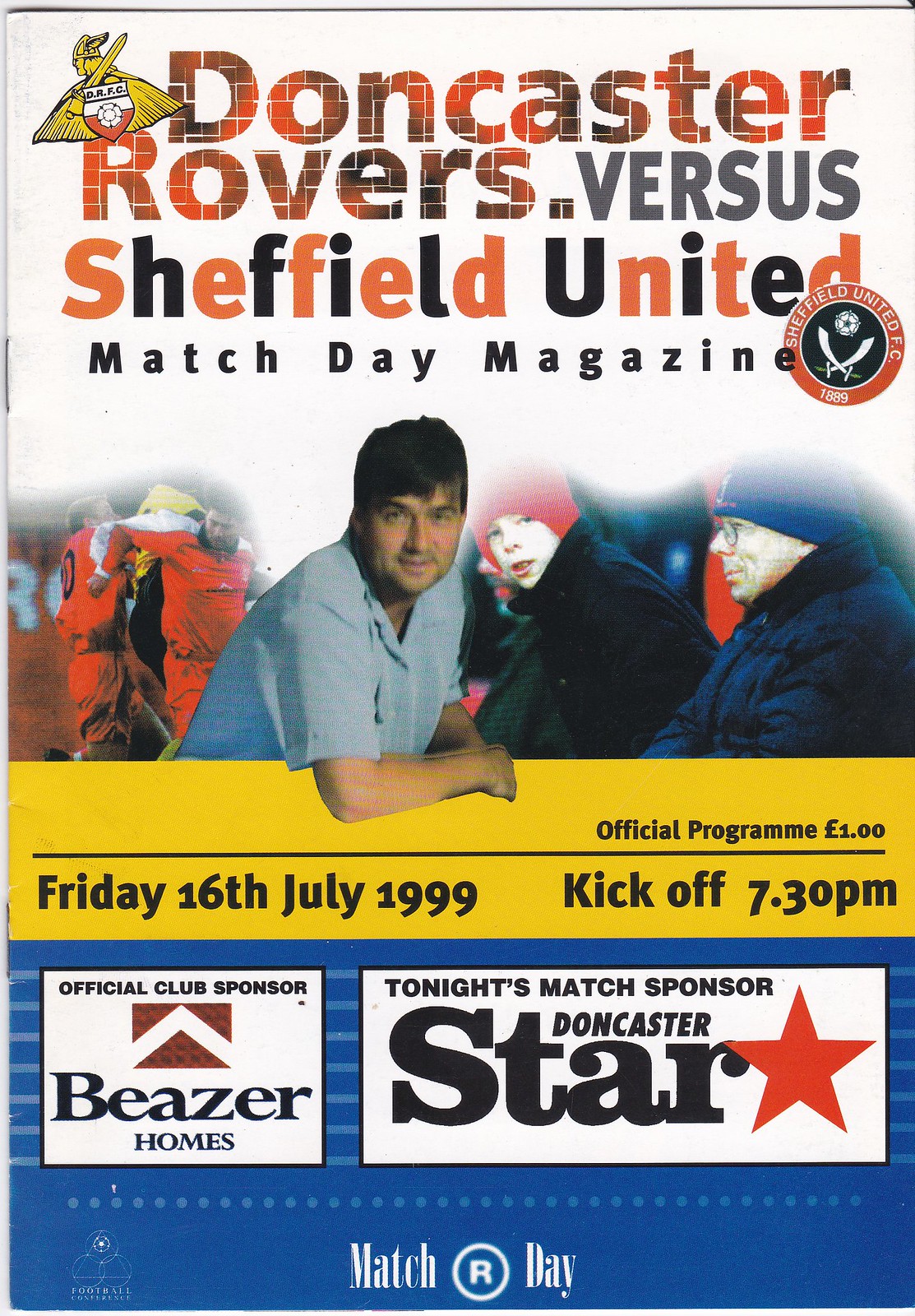This image is a detailed poster for a soccer match, prominently featuring the Doncaster Rovers versus Sheffield United. At the top, set against a white background, the text "Doncaster Rovers vs. Sheffield United" appears as if it's written on a brick wall, with "Sheffield United" alternating in red and black letters. Below that, "Match Day Magazine" is displayed in black.

Centered is a photo of a man leaning over a yellow banner, directly facing the camera, and flanked by soccer players on the left and warmly-dressed spectators on the right. The yellow banner includes black text that reads: "Friday, 16th July 1999. Official program, one pound, kickoff 7.30pm."

Beneath the banner, the background transitions to blue, featuring two white squares. The left square announces "Official Club Sponsor Beezer Homes," and the right one states, "Tonight's Match Sponsor Doncaster Star." Below these squares, in white text, it states "Match Our Day." Additionally, it's noted that Sheffield United FC was founded in 1889. The overall design clearly marks it as the cover of the official program for the match, priced at one pound.